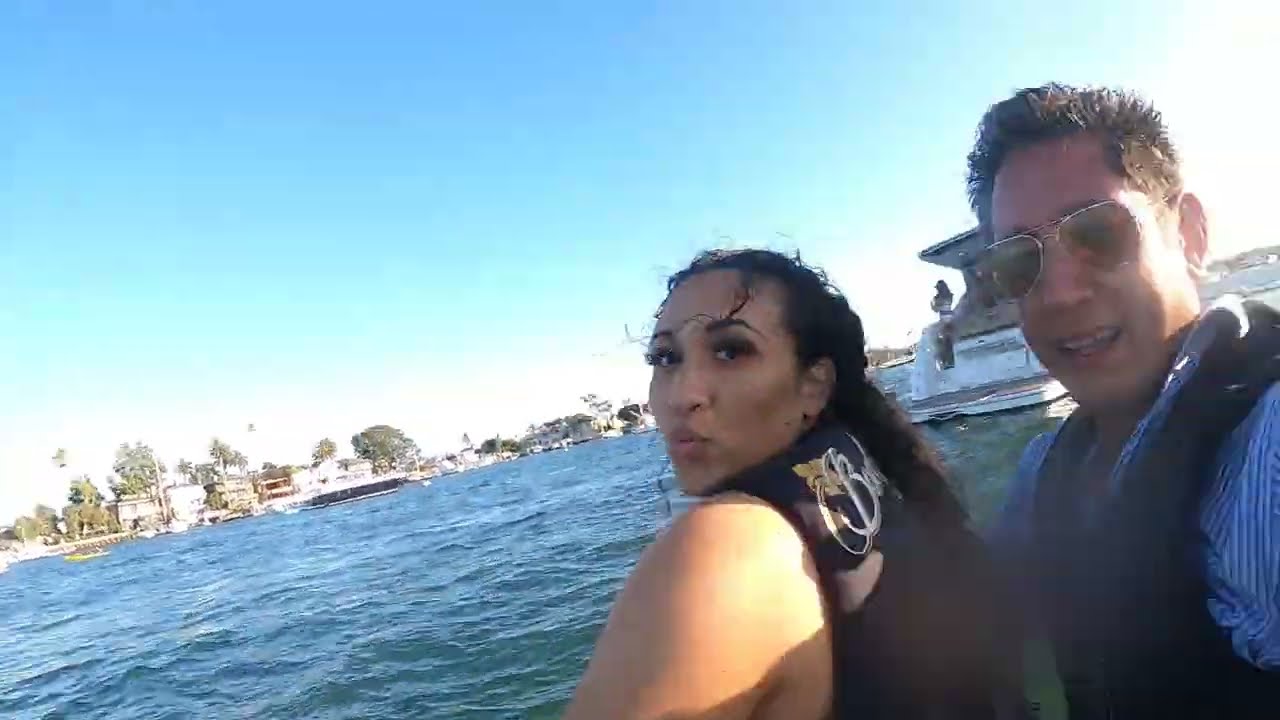In this vibrant selfie, two people dominate the right-hand side, set against a picturesque nautical backdrop. The person on the right, a man donning silver sunglasses with tan lenses, is dressed in a blue and white striped button-up shirt paired with a black life vest. Beside him is a woman with a black life vest, her curly brown or black hair neatly pulled into a ponytail. Remarkably, there is white lettering on the back of her life vest, with the letter 'B' being the only visible character. In the background, a luxurious white private yacht with a flat back is anchored. A woman in a white and black dress stands on the yacht, facing away from the camera. The left side of the image reveals a dockyard filled with private ships, all floating on a serene, light blue body of water. The scene is completed with a blue sky and distant green trees, adding a refreshing touch of nature to the aquatic setting.